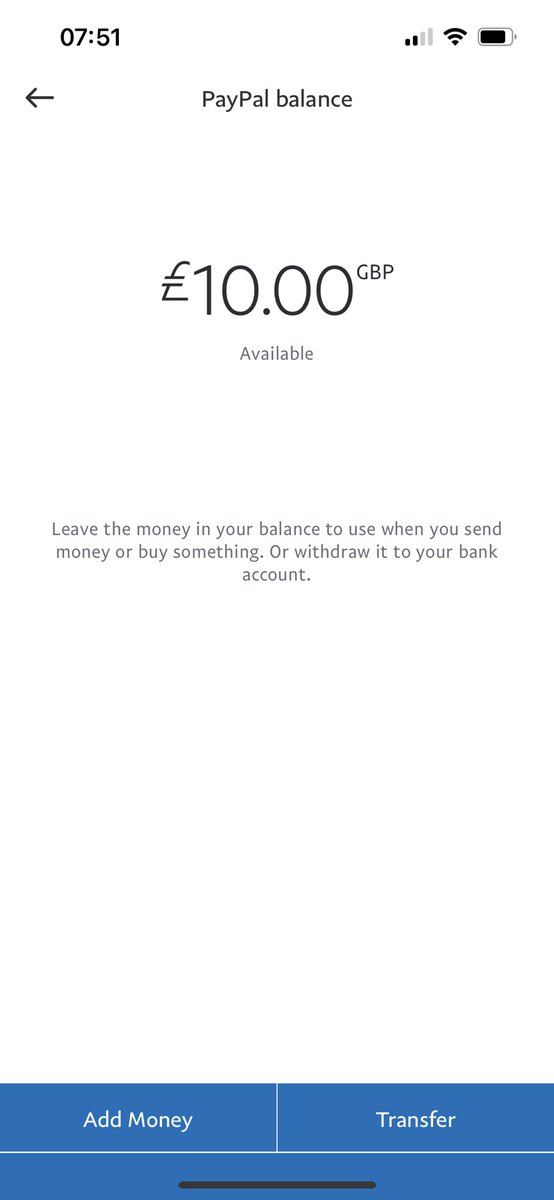In this detailed screenshot of an iPhone, taken at 7:51 AM as indicated by the time in the top-left corner, we observe various status indicators. At the top-right corner, the network signal is shown with two out of four bars, and the Wi-Fi signal strength is full with three out of three bars. Adjacent to this, we see the battery icon. 

The central part of the image displays the PayPal app interface against a white background. It shows a PayPal balance of £10 available, with the accompanying text advising the user to either leave the money in their balance for future transactions or withdraw it to their bank account. Below this information, there are action buttons including "Add Money" and "Transfer." 

At the bottom of the screen, the navigation bar features distinctly colored buttons in white, blue, and black, guiding the user through various app functions. The clean layout and specific details provide a clear snapshot of the iPhone's status and the PayPal app's functionality at that moment.